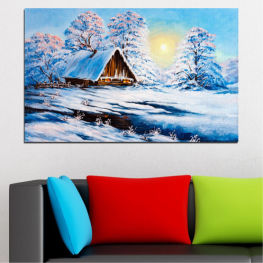A modern grayish-black leather couch with clean, angular lines is set against a white wall. Three colorful throw pillows—blue on the left, red in the center, and lime green on the right—adorn the couch. Above it hangs a large painting depicting a winter wonderland scene. The artwork features a snow-covered A-frame cottage surrounded by snowy trees, with the sun peeking through on the right side. The painting conveys a mid-century traditional style, creating a stark contrast with the modern design of the couch and pillows below.